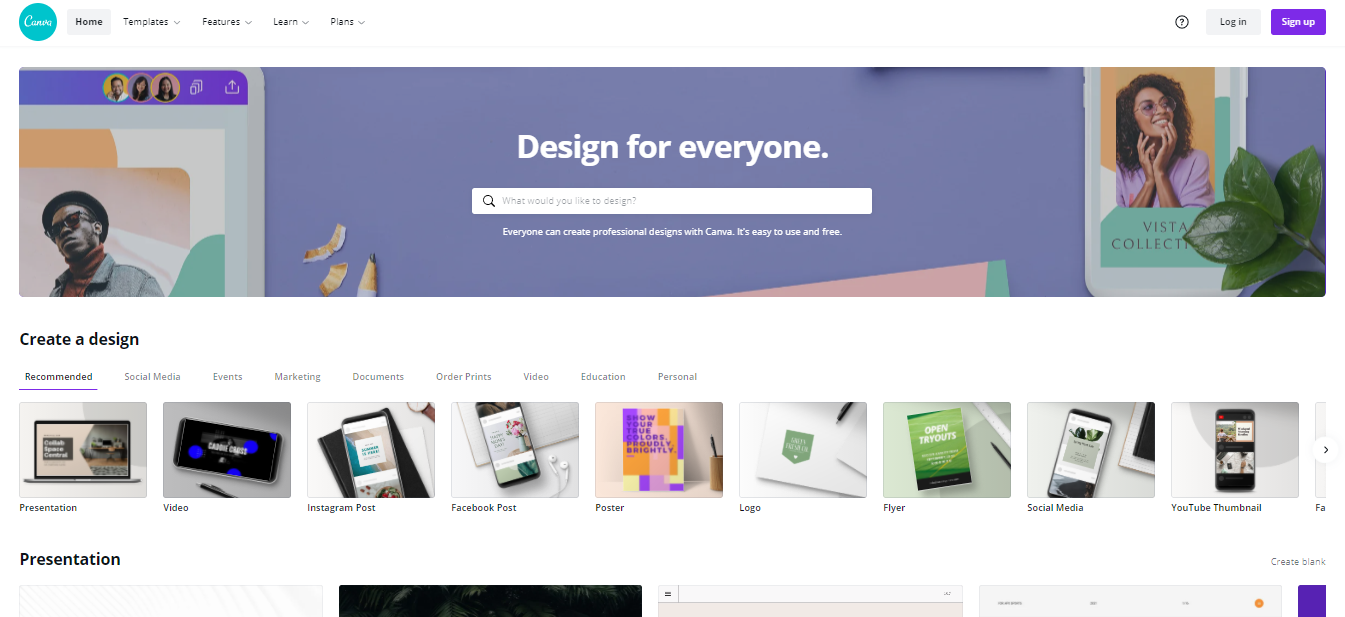The image showcases a designer's website for creating designs, featuring a blend of technology and vibrant visuals. At the top, a purple background sets a creative tone. Central to the image are two dark-skinned individuals: a man on the left and a woman on the right. Above the man are three profile pictures, adding a social element to the design experience. Below them, the text "Create a Design" invites users to explore their creativity across various devices such as a desktop computer, laptop, and phone, highlighting the platform’s versatility.

In the lower section, beneath the woman, there's a prompt to "Visit a Collection," indicating a curated selection of design examples. Among these examples, the most striking is a colorful composition in the middle, showcasing a mix of purple, orange, and lighter shades, resembling an artistic workstation. The collection also includes black-and-white images, with a particular one featuring blue dots standing out for its minimalist aesthetic. Another noteworthy design is an eye-catching lime green image, adding a fresh and vibrant touch to the assortment.